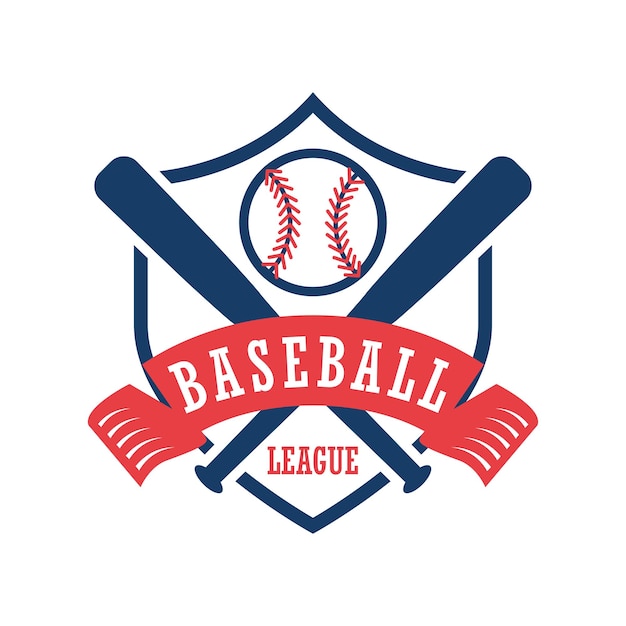The image features a vibrant, animated logo on a white background with no border. At its core, the design is centered around a dark blue shield, which serves as the primary shape. Dominating the upper section is a baseball, outlined in blue with distinct red stitching, positioned prominently at the top of the shield. Central to the design and crossing each other diagonally are two dark blue baseball bats, creating a striking focal point. Beneath the baseball and intersecting the bats is a red banner that spans across the width of the shield. Emblazoned on the banner in bold, white, capitalized letters is the word "BASEBALL." At the bottom tip of the shield, snugly fitting between the handles of the crossed bats, is the word "LEAGUE," also in bold red, capitalized text. This meticulously crafted logo is likely intended for a baseball league, possibly as a mock-up for community-level teams, providing a clear and vivid representation that could be used for promotional materials or merchandise.